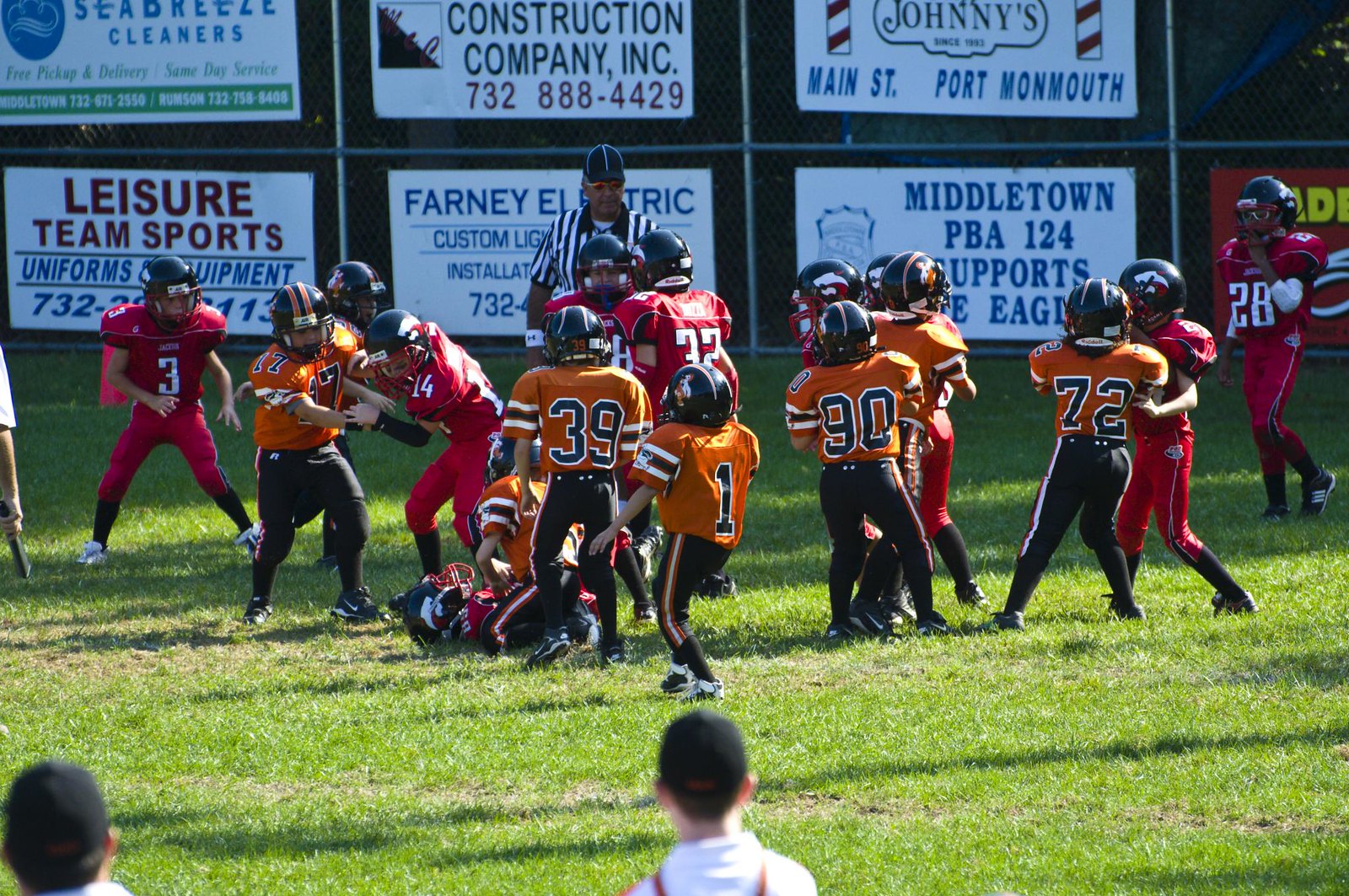The image captures a lively youth football game on a lush green grass field. Two teams are competing, with players in either orange jerseys with black pants and helmets, or red jerseys with matching pants and helmets. One red-uniformed player lies on the ground, seemingly tackled by an opponent in orange. Other players are engaged in a close encounter nearby, while a referee looks on from the background. The scene is vibrant with activity and youthful energy. Several white advertising banners, affixed to a large chain-link fence in the background, display local sponsors, including Scadrille Cleaners, Construction Company Inc., Johnny's Barbershop with iconic barber poles, Leisure Team Sports Uniforms and Equipment, Farney Electric, and Middletown PBA 124 Supports Little League. Additionally, two children wearing black baseball caps are visible in the foreground, observing the game intently.